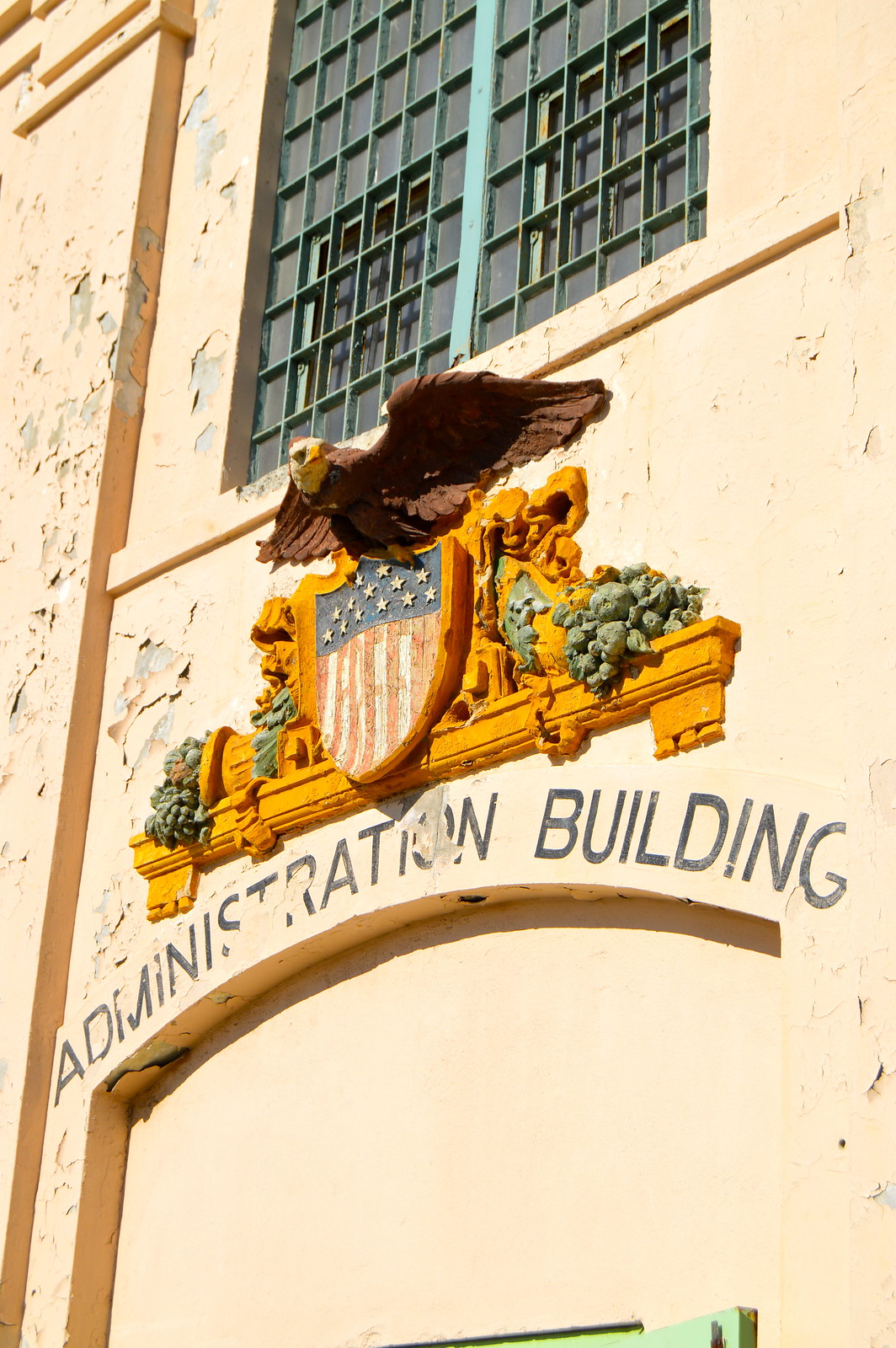This image features a detailed view of the aging facade of an Administration Building, most likely located in the United States. Dominating the space above an arched entryway is a weathered relief of a bald eagle with spread wings, perched atop a shield resembling the American flag. The flag on the shield is distinctively styled with vertical stripes and an arrangement of stars that likely represent the original 13 colonies. Flanking the shield are reliefs of grapevines, adding a touch of nature to the otherwise institutional facade.

The entire surface of the beige stucco wall is marred by extensive peeling and cracking, hinting at the building’s considerable age and possibly indicating it could be abandoned or in serious need of maintenance. Above the eagle and shield ensemble, a barred window with dark panes adds to the sense of neglect, with cross-hatched bars guarding the glass.

Below this patriotic insignia, the words "Administration Building" are inscribed in capital letters, yet the text is faded, blending into the chipped and crumbling stucco. The image captures the upper section of the wall in a vertical format, tapering down to an arched structure where the photograph hints at a green door barely visible at the frame’s edge. The various elements—the architectural details, the cracking facade, and the suggestive symbols of American heritage—collectively narrate a story of a once-prominent building now succumbing to the ravages of time.